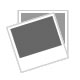The back cover of the DVD for "The Wizard of Gore" features large white text with red accents that make it appear as if blood is dripping down the words, spelling out the title "The Wizard of Gore." Beneath this, in smaller red text, is the tagline: "Is it magic or wholesale slaughter?" The cover has a black background and includes a descriptive blurb about the movie. The first paragraph introduces Montag the Magnificent, a seedy small-time magician played by Ray Sager, who hypnotizes pretty young women from the audience to participate in his shocking stage act, mutilating them in grand illusions, including being cut in half with a chainsaw, drilled through the stomach with a giant punch press, and having a metal spike driven through their head. Additionally, there is a smaller thumbnail image showing a magician standing over an open coffin with a woman inside, placed next to flowers in a shallow grave. The cover also lists the actors and production crew in the middle section. The DVD case appears sealed in plastic and sits on a wooden surface, with a barcode visible in the top right corner.